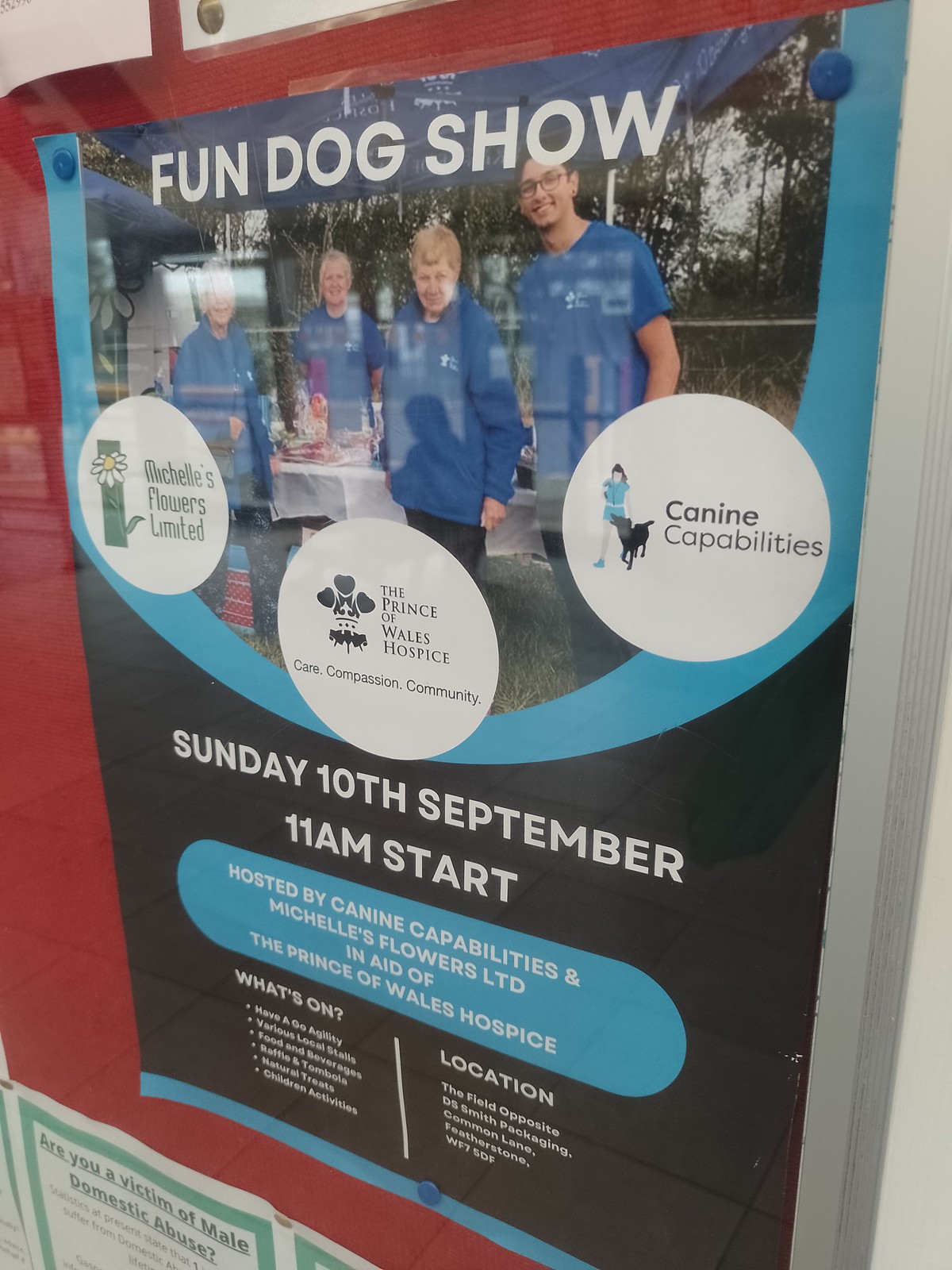This photograph captures a colorful advertisement poster prominently displayed on a red wall. The main title at the top of the poster reads "Fun Dog Show" in white text. Below the title is an image featuring four people dressed in blue shirts. Among them, an older man stands to the left, two older women in the middle, and a younger, taller man with black hair on the right, all smiling. Beneath this image are three white circular logos: the left one reads "Michelle's Flowers Ltd.," the center one states "The Prince of Wales Hospice," and the right one says "Canine Capabilities."

Further down, the poster announces the event details: "Sunday, 10th September, 11 a.m. start," followed by a smaller text segment within a blue pill-shaped banner that reads, "Hosted by Canine Capabilities and Michelle's Flowers Ltd. in aid of the Prince of Wales Hospice." The lower section of the poster features a "What's On?" list with six bullet points, and to the right, information on the event's location. Surrounding the main poster are several green flyers and another smaller white poster about male domestic abuse with bold, black underlined text, which is partially legible.